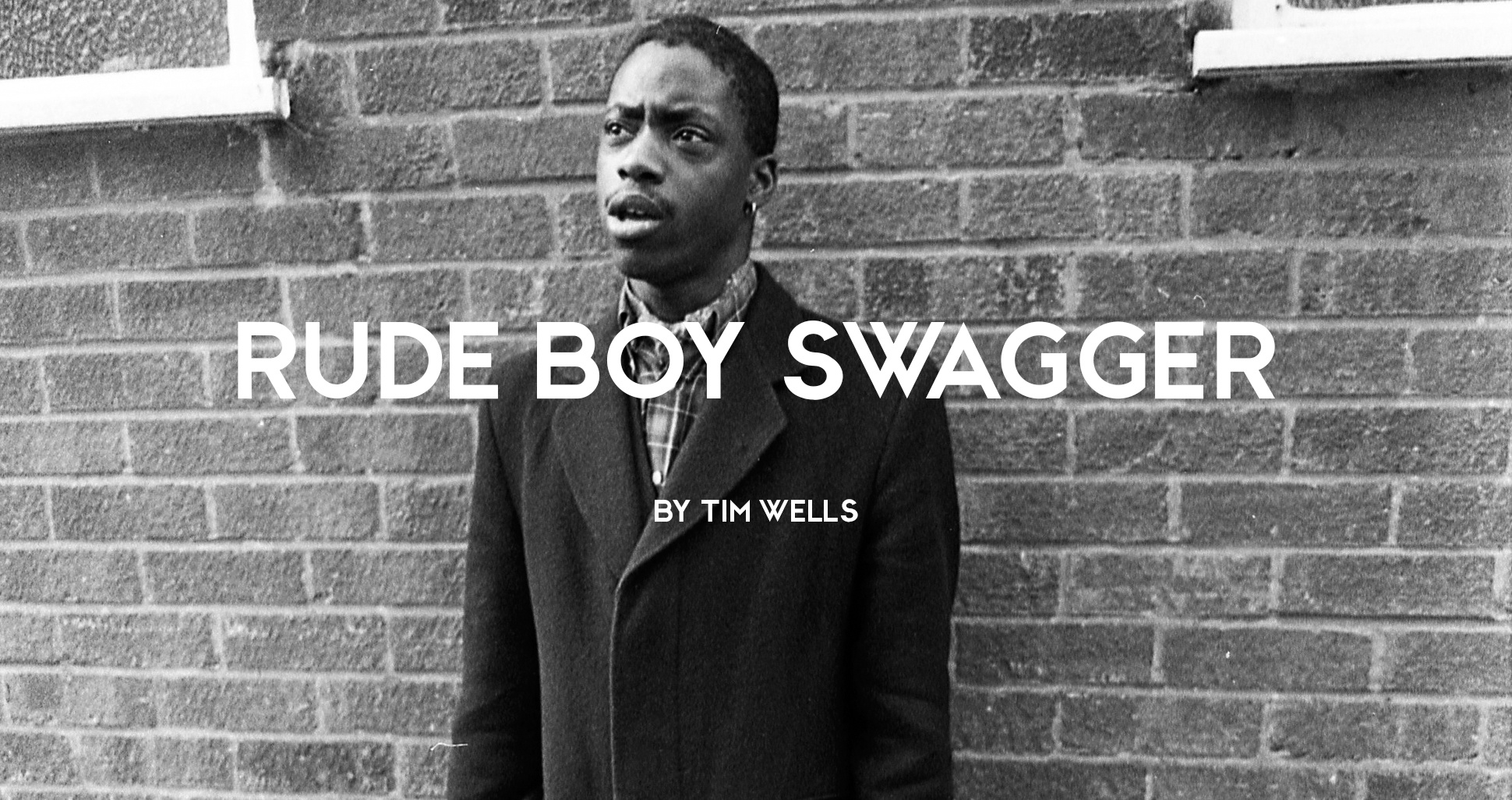This black-and-white photograph, titled "Rude Boy Swagger" by Tim Wells in bold white capital letters, showcases a young African-American man standing against a brick wall, presumably in front of a building. The man's intense expression, with a slightly open mouth and furrowed brow, suggests a look of disbelief or annoyance. He has short dark hair and wears an earring. Dressed in a formal-looking wool overcoat over a less formal plaid button-up shirt, he appears bundled up for the outdoors. The image subtly captures the building's windows behind him, adding to the urban setting ambiance.